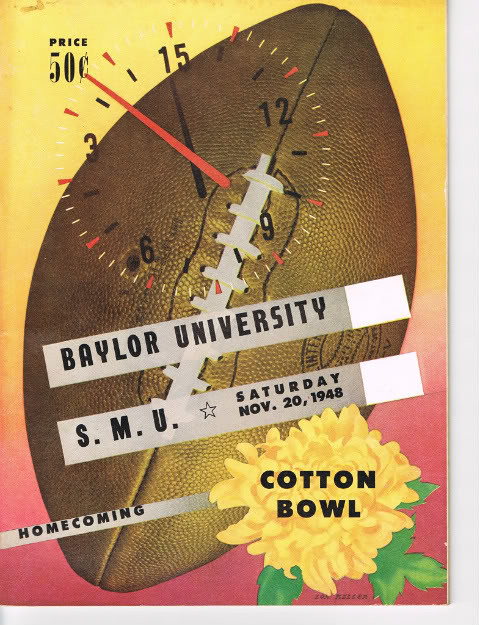This is a colorful, vintage poster advertising a college football game, specifically the Cotton Bowl, priced at 50 cents and dating back to Saturday, November 20, 1948. The background of the poster features a gradient that transitions from yellow at the top to pink and red hues towards the bottom. Dominating the center is a brown, old-school football, slightly angled, with a superimposed clock displaying the numbers 3, 6, 9, and 12, along with red and black clock hands. Above the football, in a semi-transparent white block, the black text reads "Baylor University" at an angle, followed by "SMU," both teams part of the highlighted event. Adding to the nostalgic theme, a yellow flower with green leaves sits in the bottom-right corner with the bold text "Cotton Bowl" inscribed across it. The poster also indicates this is a homecoming game, giving further significance to the event.